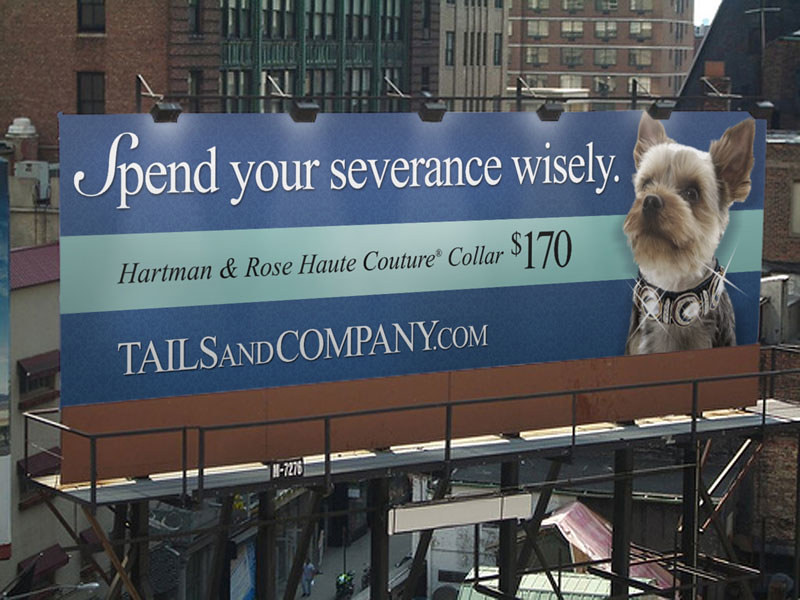In the midst of a bustling daytime cityscape, a striking billboard stands illuminated against the sky, though it hardly needs the overhead lights given the bright daylight. The billboard, perched above what appears to be a gritty alleyway lined with dilapidated buildings, is emblazoned with bold white text commanding, "Spend your severance wisely." Just below, in a contrasting black font, it advertises "Hartman and Rowe’s Hot Couture Collar, $170." Beneath this, the call-to-action, "tailsandcompany.com," is prominently displayed. Dominating the right side of the billboard is an eye-catching photograph of a small Yorkshire Terrier, its head turned upward, showcasing a dazzling, jewel-encrusted collar that sparkles brilliantly. The background reveals tall apartment buildings, framing the scene and emphasizing the juxtaposition of luxury advertising against a less affluent urban setting.